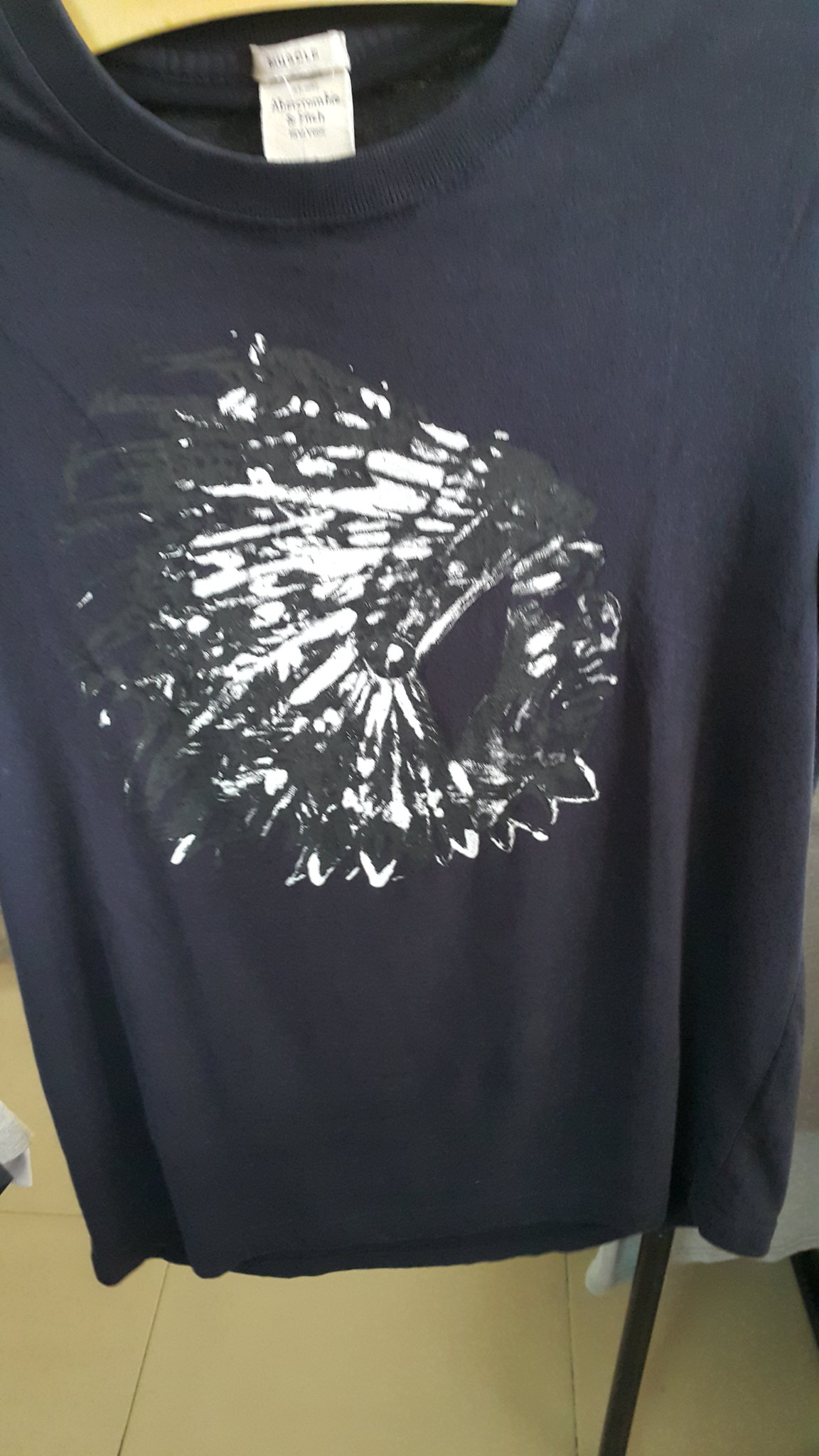This image depicts a retail setting, likely a store, indicated by the visible hangers and a beige, public space-style tile floor. At the forefront is a navy blue graphic t-shirt prominently featuring the Abercrombie & Fitch label. The shirt's central design includes a black and white illustration resembling large feathers, possibly reminiscent of peacock feathers, giving it a distinct, stylish look. The t-shirt hangs from a light brown hanger on a rack, alongside additional clothing items in the background. While the exact size of the shirt is unclear due to some blurriness in the image, the Abercrombie & Fitch branding is clearly noticeable.